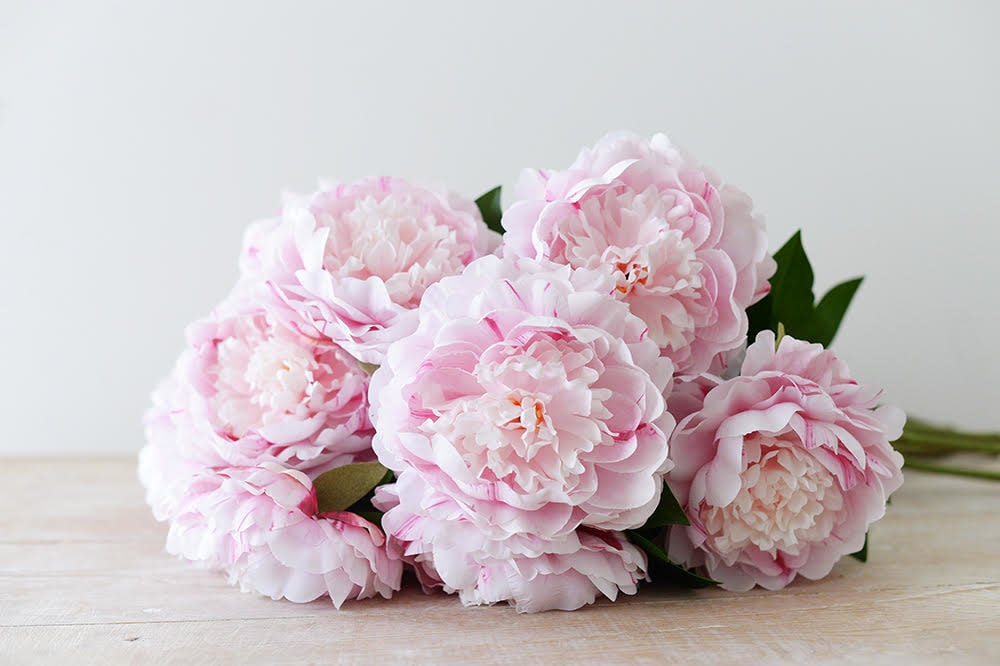A delicate arrangement of seven pale pink carnations is elegantly displayed on a light wooden table, bathed in bright natural light from the left. The flowers are laid on their sides, facing the camera, revealing their full, rounded blooms and innermost white buds. The blooms, varying from light pink to hints of darker pink, are positioned such that three flowers line up on the left, three in the center, and one to the right. The stems and sparse green leaves, though mostly obscured by the flowers, are faintly visible on the right, blending into a slightly blurred background. The intense lighting accentuates the contrast against the off-white wall behind the arrangement, creating a pastel-like ambiance. The image is suffused with a pastel purple hue, giving it a soft and dreamy quality.